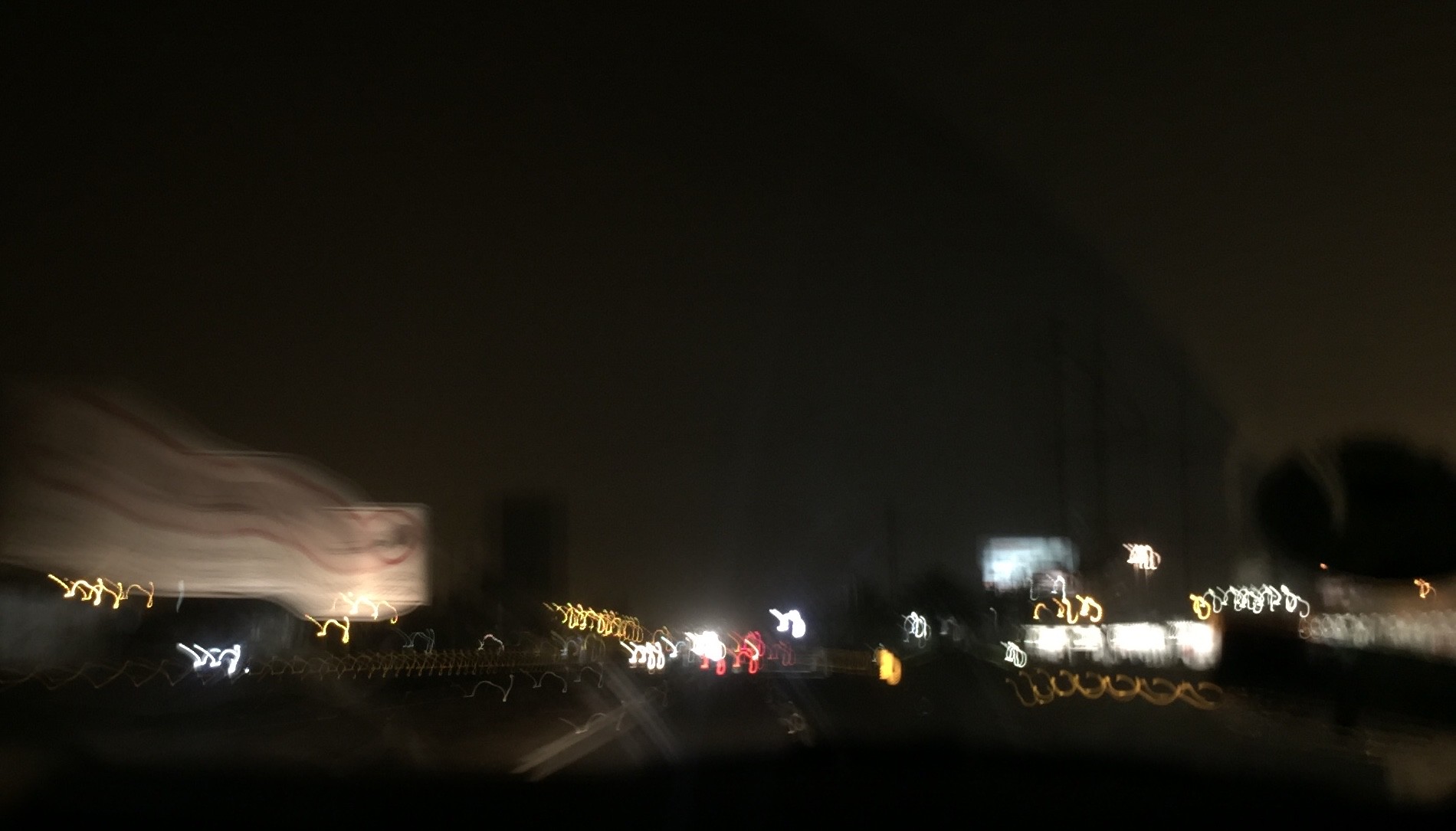A blurred nighttime scene depicting a street, shrouded in near-total darkness. The image is heavily obscured, with only various streaks of moving lights breaking through the murkiness. On the left-hand side, a distorted street sign appears, painted white with a black symbol encircled in red, which looks like a wavering ribbon due to the unsteady camera. Across the frame, there are chaotic spirals of multicolored lights—yellow, white, and red—resembling the headlights or taillights of passing vehicles and possibly lit traffic signs, creating a surreal, almost abstract visual effect.